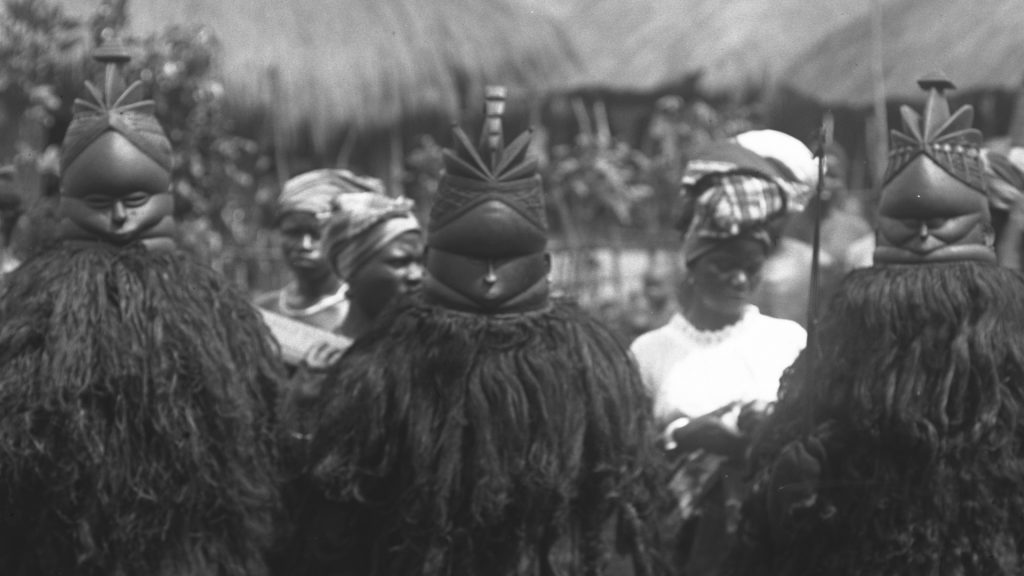This black-and-white photograph, likely over 50 years old, depicts three individuals in the foreground and three women in the background. The foreground features three people adorned in elaborate tribal masks and wearing long, furry robes that could be fashioned from animal fur or naturally occurring fibers. These masks, possibly carved from wood or molded from metal, have a matte finish and human-like facial features including high, narrow cheekbones, small noses, and tiny eye indentations. Atop each mask sits a distinctive disc arrangement, resembling the shape of a pineapple. 

In the background, three women with dark skin are visible. One woman is dressed in a white top while the other two wear off-the-shoulder, light-colored blouses. One of these women sports a metallic necklace. Each woman has patterned fabric wraps tied around their heads, which might be colorful if seen in color. The background also contains blurry greenery, suggesting the setting might be amidst lush vegetation, possibly in Africa.